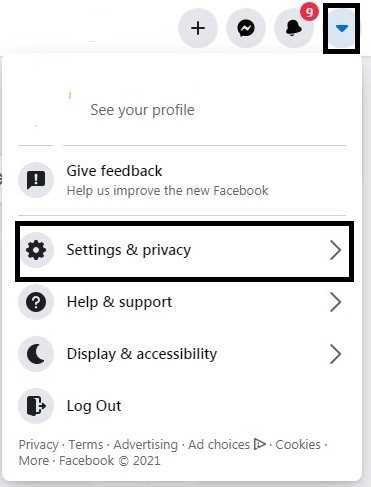The image displays a simplified profile menu interface on a white background. At the top, a section labeled "See Your Profile" is prominently featured in gray text, separated by a horizontal line. Below this section are various options:

1. **Give Feedback:** 
   - Text: "Help us improve the new Facebook."
   - Icon: A circle featuring a chat bubble with an exclamation point in the middle.

A second horizontal line divides the interface, followed by four key sections, each with corresponding icons on the left and arrows on the right:

2. **Settings & Privacy:**
   - Icon: A cogwheel.

3. **Help & Support:**
   - Icon: A question mark.

4. **Display & Accessibility:**
   - Icon: A moon.

5. **Log Out:**
   - Icon: An open door.

At the bottom of these sections, smaller gray text lists links for "Privacy," "Terms," "Advertising," "AdChoices" — each followed by a right-arrow — and the line "More," followed by "Facebook" and the copyright symbol, "© 2021."

Above the entire menu, there are three user interface icons:

- A plus sign.
- A speech bubble with a lightning bolt.
- An alarm bell with the number "9" indicating notifications.

To the far right, there is a down-pointing blue arrow outlined in black. Notably, the "Settings & Privacy" section is outlined in black, emphasizing its importance.